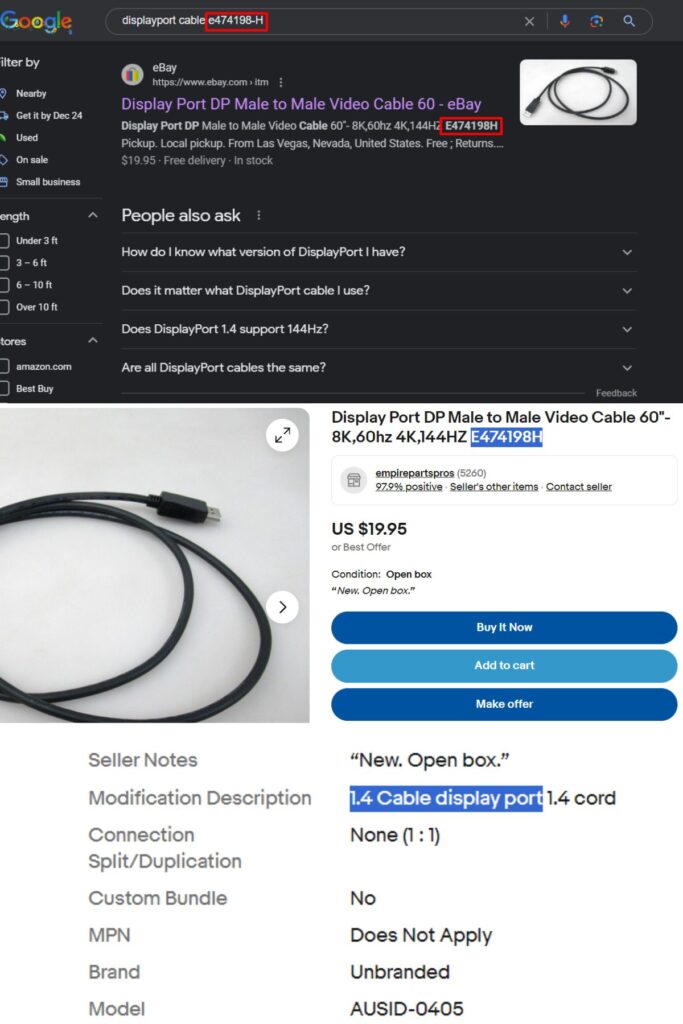A person is actively searching for a DisplayPort cable online. The browser is open to Google with the search term "DisplayPort DP male-to-male video cable" prominently displayed. The top search result shows an eBay listing featuring a DisplayPort male-to-male video cable capable of 8K resolution at 60Hz. The cable is listed for $19.95 and is in an open-box condition. On the eBay page, there are options to buy it now, add it to the cart, or make an offer. Additional details include that the item is unbranded, with no custom model number or specific NPM mentioned. The potential buyer appears to be weighing their options, considering either purchasing it immediately or looking elsewhere for a similar product.